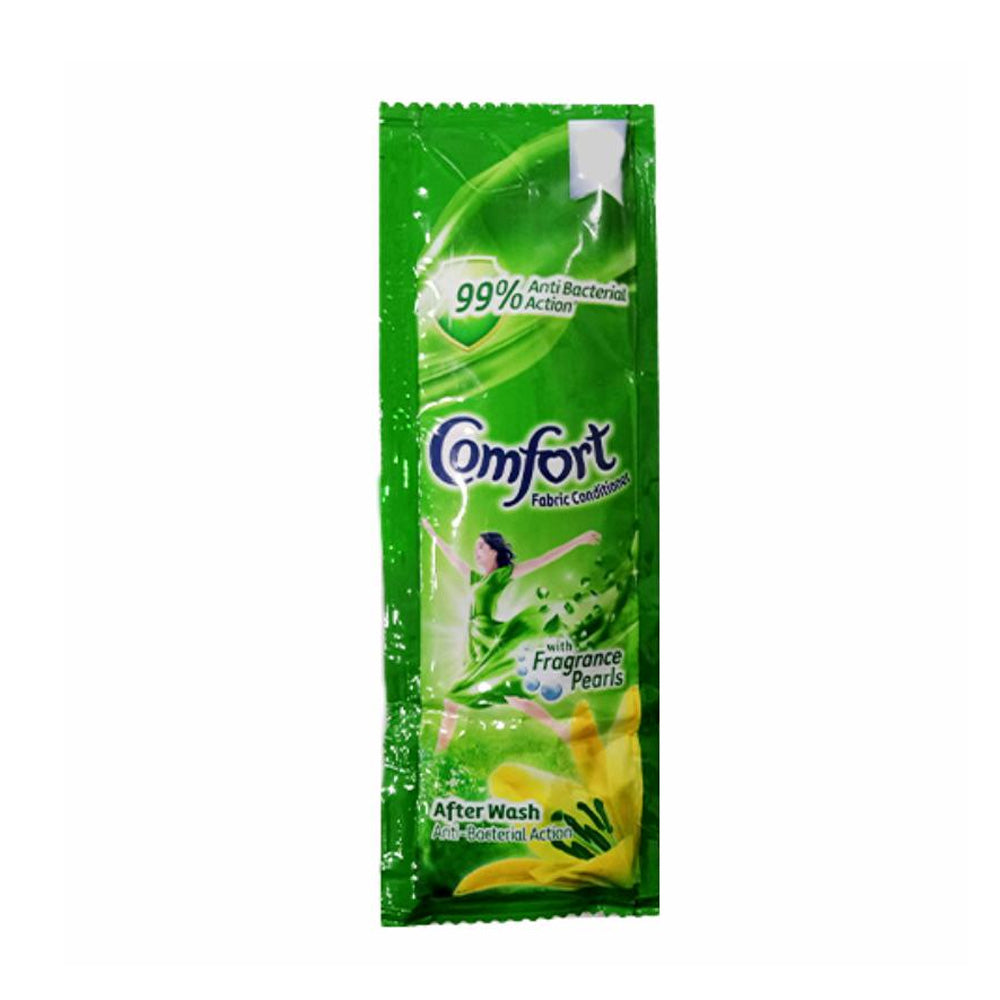This photograph captures a green plastic packet of Comfort Fabric Conditioner with a pristine white background. The prominently flat and wrinkled packet, resembling the texture of a ketchup packet, features corrugations on the top and bottom indicating where it can be opened. The upper right-hand corner of the packet displays a white square with "99% Antibacterial Action" emblazoned in front of a green shield. In the center of the package, "Comfort Fabric Conditioner" is written in dark blue font, with a heart-shaped "O" adding a touch of softness to the brand name. Below the product name, a joyful woman in a green dress is depicted frolicking outdoors, with green objects extending from her dress like flower petals. The phrase "With Fragrance Pearls" is shown above a pearl ring sequence. Dominating the foreground is a large yellow flower, above which "After Wash Antibacterial Action" is declared. The packet has been opened and used, indicating its prior utility, and it rests unaccompanied on a surface without any other objects in the background. The color palette of the packet includes shades of green, blue, yellow, and white.